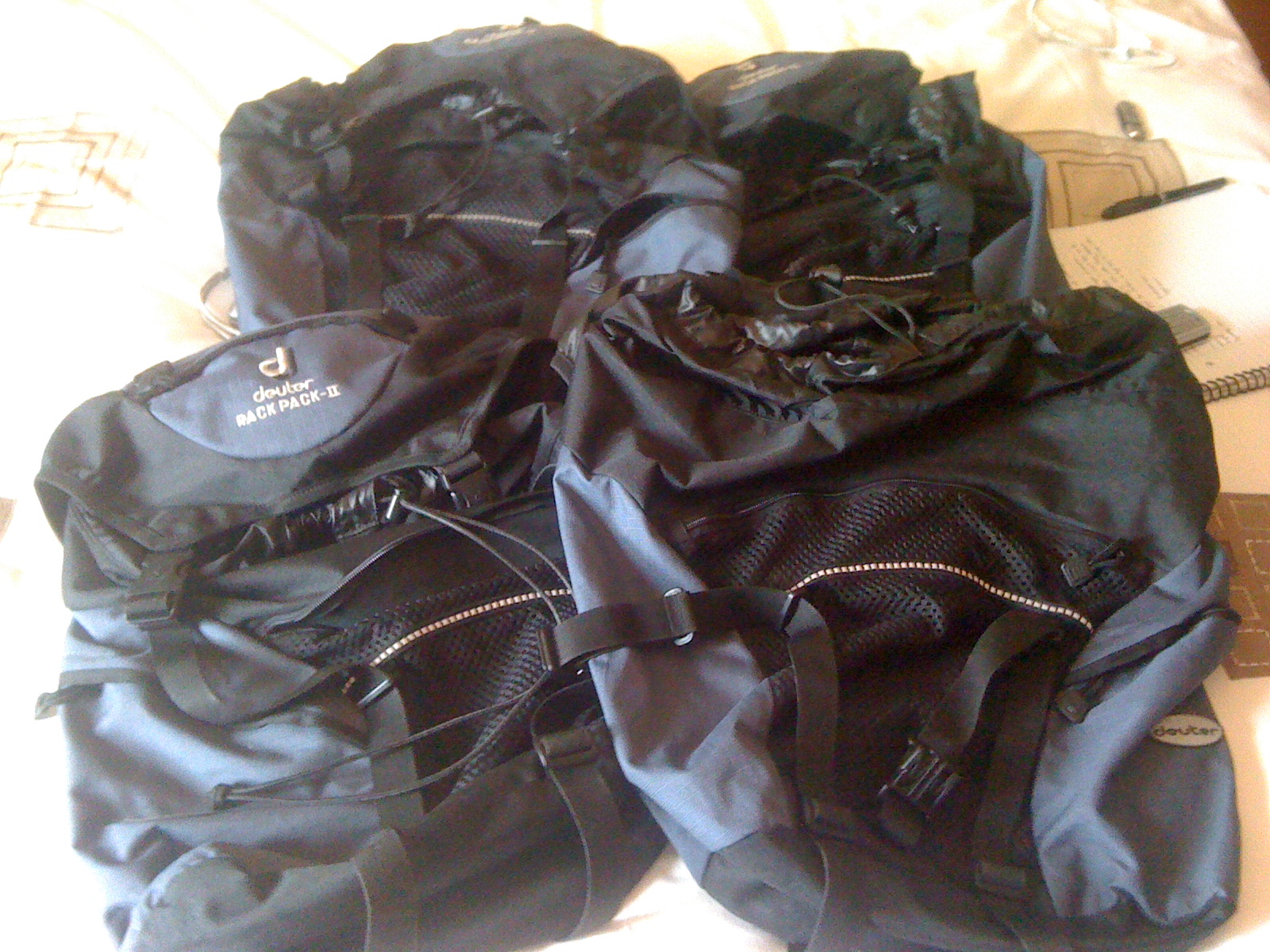In this horizontal close-up image, we see a group of three Deuter backpacks with the model name "Backpack 2" prominently displayed. The backpacks have dark blue and black colors, with the brand’s distinctive large gold letter "D" and "DEUTER" inscribed below it on the flap. These backpacks have multiple black straps, a black net bag in the front, and several compartments for storage, making them ideal for college students, hikers, or backpackers. They are arranged in a triangular formation on a bed in a well-lit room, along with a cylindrical black duffle bag featuring black cords and straps. A notebook and pen are also spotted on the bed, suggesting preparation for an upcoming trip.